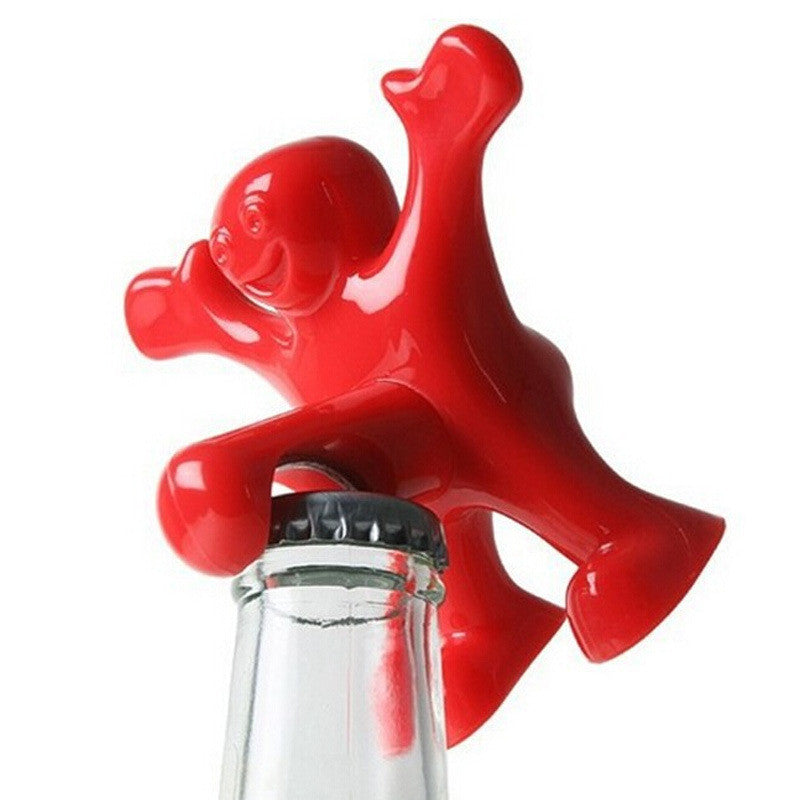In this square image, the background is completely white, highlighting a striking and unusual bottle opener attached to the neck of a glass bottle. The bottle features a silver, ridged metal bottle cap, partially obscured by a bizarre, shiny red plastic object shaped like a character. This character appears to be bald with a large, smiling face and big eyes. Its arms, which resemble mittens, are stretched upward, and its legs, along with thick feet and a small butt, are splayed outwards. A red plastic protrusion extends from the middle of the character's body downward toward the left, securely wedging itself around the bottle cap. The overall effect is one of whimsy and peculiarity, making the object appear lively and engaging against the stark white backdrop.